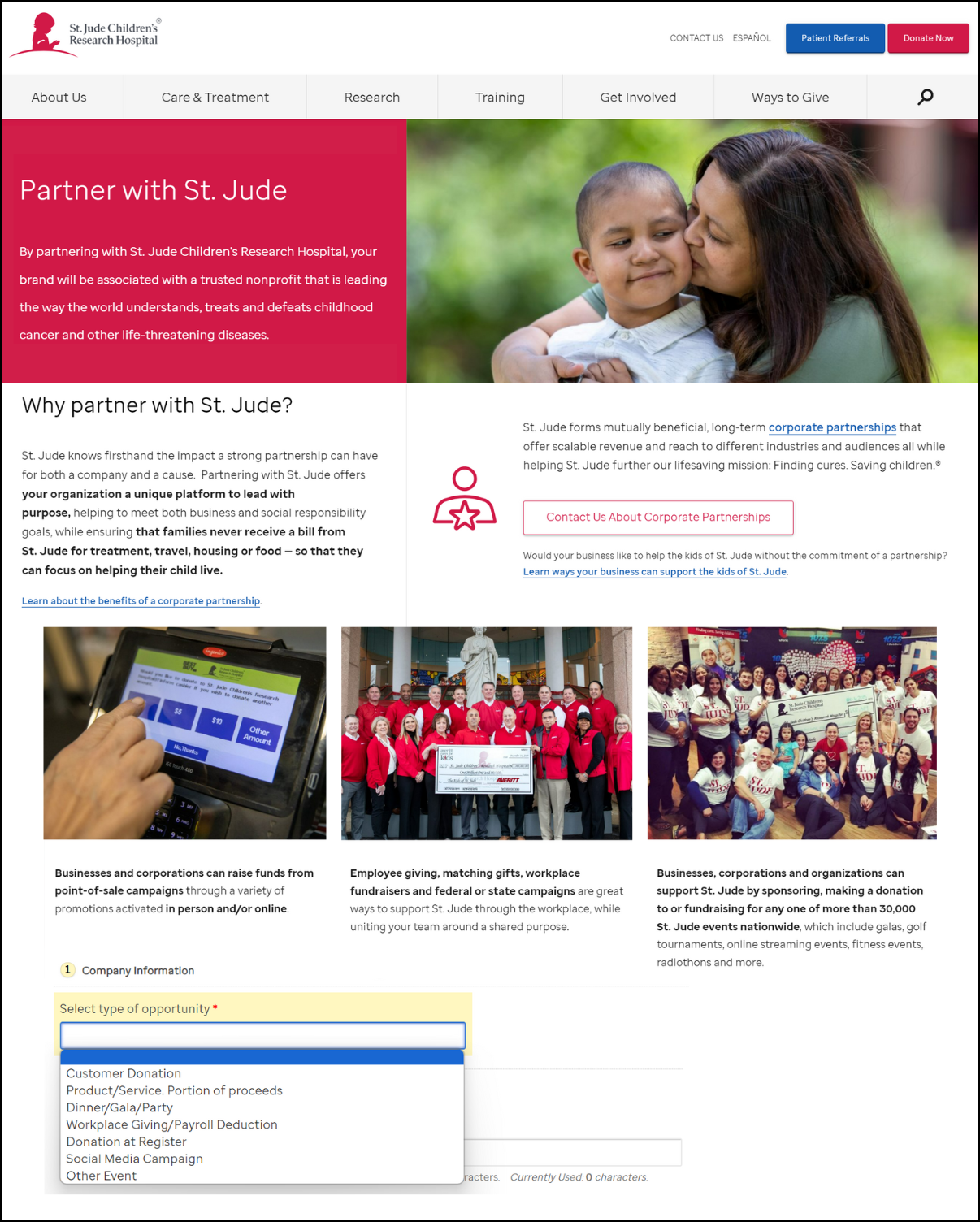This image appears to be a screenshot of the homepage from the website of St. Jude Children's Research Hospital, designed for display on a tablet. At the top left, a pink banner states "Partner with St. Jude," next to which is a touching photo of a Mexican woman in a sage green shirt hugging and kissing a young boy with thin black hair, likely undergoing cancer treatment. The banner reads, "Partner with St. Jude. By partnering with St. Jude Children's Research Hospital, your brand will be associated with and trusted by a nonprofit that is leading the way the world understands, treats, and defeats childhood cancer and other life-threatening diseases."

Below this, a section titled "Why Partner with St. Jude" explains in detail why it is beneficial to support the institution, highlighted in small but informative text. Adjacent to this text are three images: the first one depicts a machine, resembling a credit card terminal, with a hand pressing a button. The middle image features two rows of about 20 people in total, all wearing red shirts and holding a large donation check. The last image shows a group of approximately 20-30 people, some standing and some sitting, likely St. Jude supporters or staff members, wearing shirts that possibly read "St. Jude." Each of these images has short descriptive blurbs beneath them. At the very bottom of the page, there is a drop-down menu labeled "Select Type of Opportunity," indicating various ways supporters can get involved.